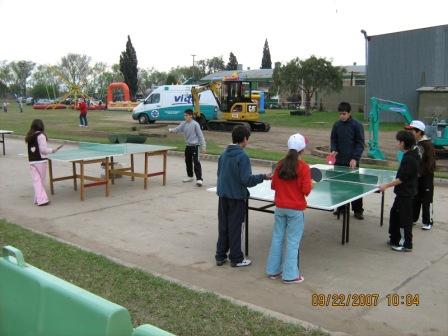In this outdoor, daytime photograph taken on an overcast day, we see two ping pong tables set up on a concrete pathway within a green field, flanked by various structures and activity. The foreground is dominated by a ping pong table to the right, surrounded by five children, predominantly of Asian descent. Two of these children, a boy and a girl, face the camera as they engage in the game, while two other kids have their backs to the camera. A tall boy dressed in black is seen with a red paddle, and beside him stands another boy in black with a white baseball cap tipped in red. The opposing players include a boy in a blue sweatshirt, blue joggers, and white trainers, and a girl wearing a red jumper, blue jeans, and white pumps with a red-tipped cap. There is also a spectator, dressed entirely in black, standing to the side, possibly acting as a line judge.

Slightly behind this table to the left, another ping pong table hosts a game between a young girl in pink trousers and a black jacket with pink sleeves, and a boy clad in a grey sweatshirt, black trousers, and white shoes. Towards the background, there's a prominent CAT-branded yellow construction mini backhoe on tracks. Adjacent to this equipment is a white van with unreadable text, and further back, there appears to be a festival scene featuring a gazebo, a parking lot, and possibly a colorful children's play area.

In the upper right of the photograph, a timestamp in yellow lettering reads "09-22-2007" at "10:04".